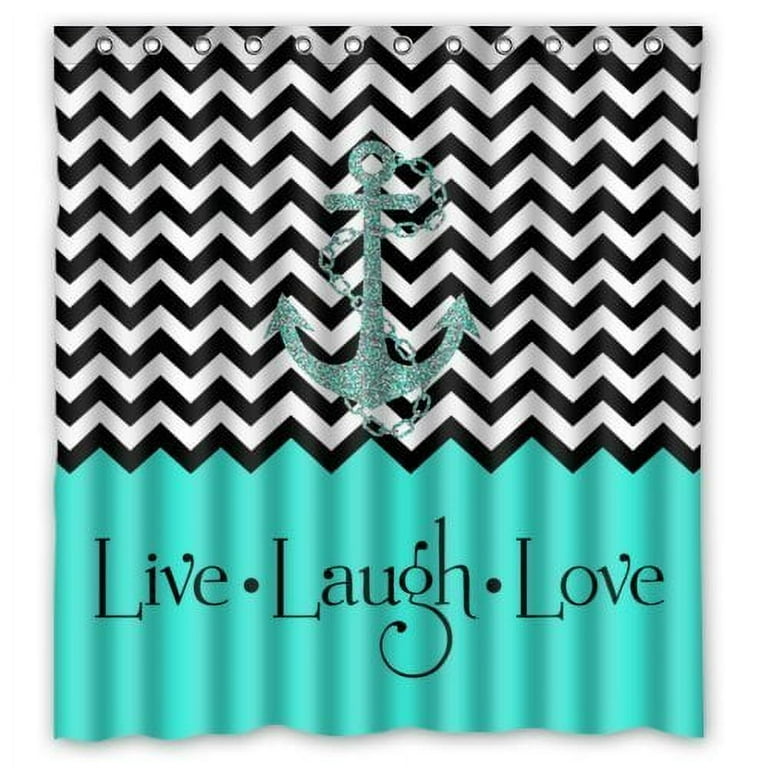This image portrays a vertically rectangular shower curtain, predominantly divided into two striking sections. The top two-thirds feature bold, black-and-white zigzag stripes running horizontally, creating a visually engaging pattern. In the center of this zigzag section is a blue and grey, glittery anchor with a chain intricately wrapped around it, adding a touch of maritime charm. The bottom third of the curtain is a vibrant turquoise background, upon which the phrase "LIVE. LAUGH. LOVE." is prominently displayed in large black letters. At the very top, white circles within silver eyelets are visible, indicating where the curtain would be hung using hooks. The curtain has a subtle gray shadow border but no distinct background, making the design elements stand out vividly.